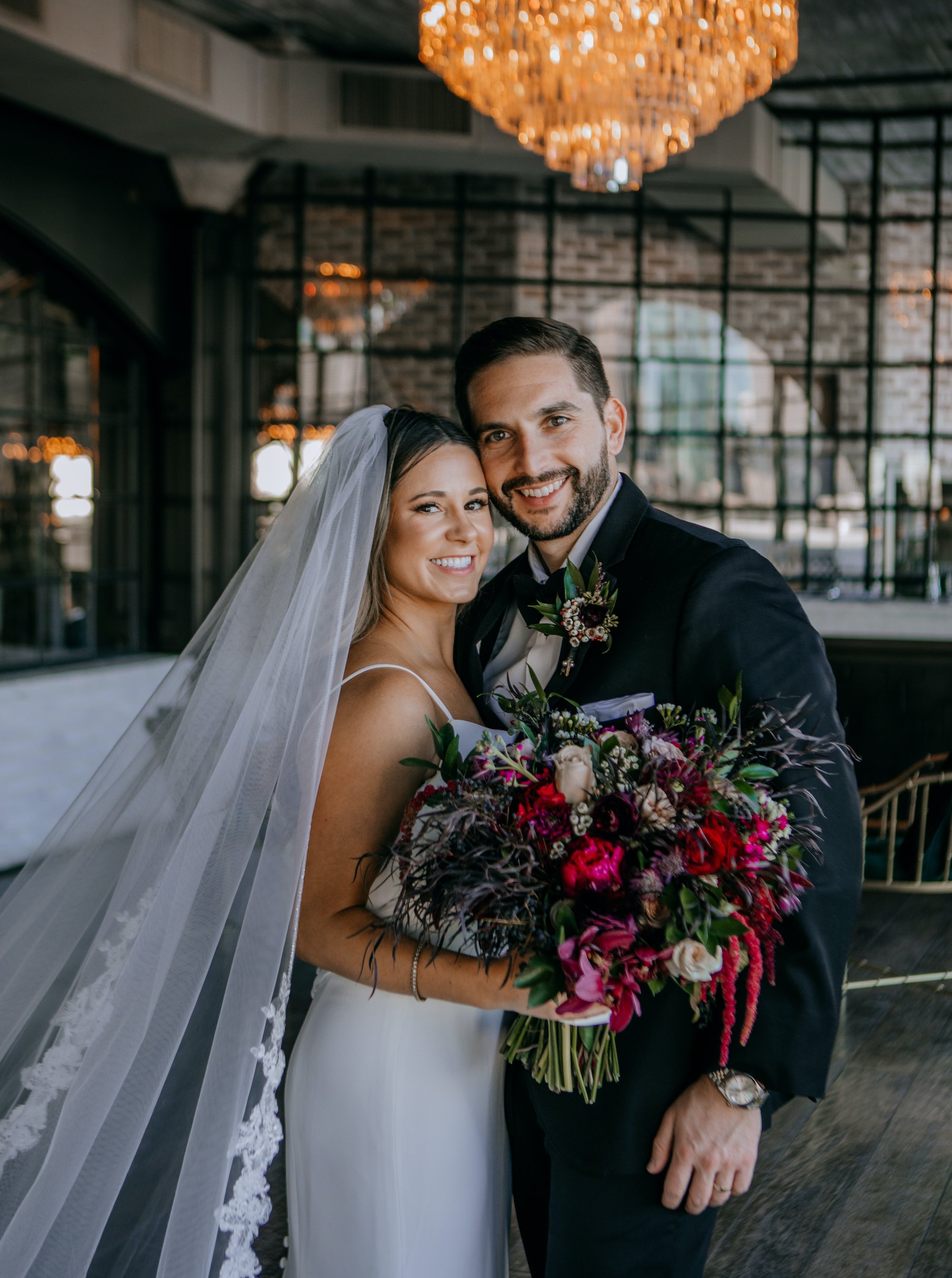In this photograph, a newlywed couple poses cheek to cheek, radiating happiness on their special day. The bride is adorned in an elegant white bridal gown complemented by a long, flowing veil. She clutches a large, vibrant bouquet of flowers, adding a burst of color to her ensemble. The groom, slightly taller than his bride, sports short dark hair and a meticulously groomed mustache and beard. Dressed in a sharp black jacket over a light blue shirt, he too smiles warmly at the camera.

The setting appears to be a rustic venue, possibly a restaurant or event room. The floor is made of rough-hewn gray wooden planks, which add a charming, rugged touch to the scene. In the background, a sofa is visible, suggesting a cozy, intimate environment. Behind the couple is a wall of windows revealing more of the venue, including some lights, red brick walls, and a few other guests, hinting at a larger celebration taking place.